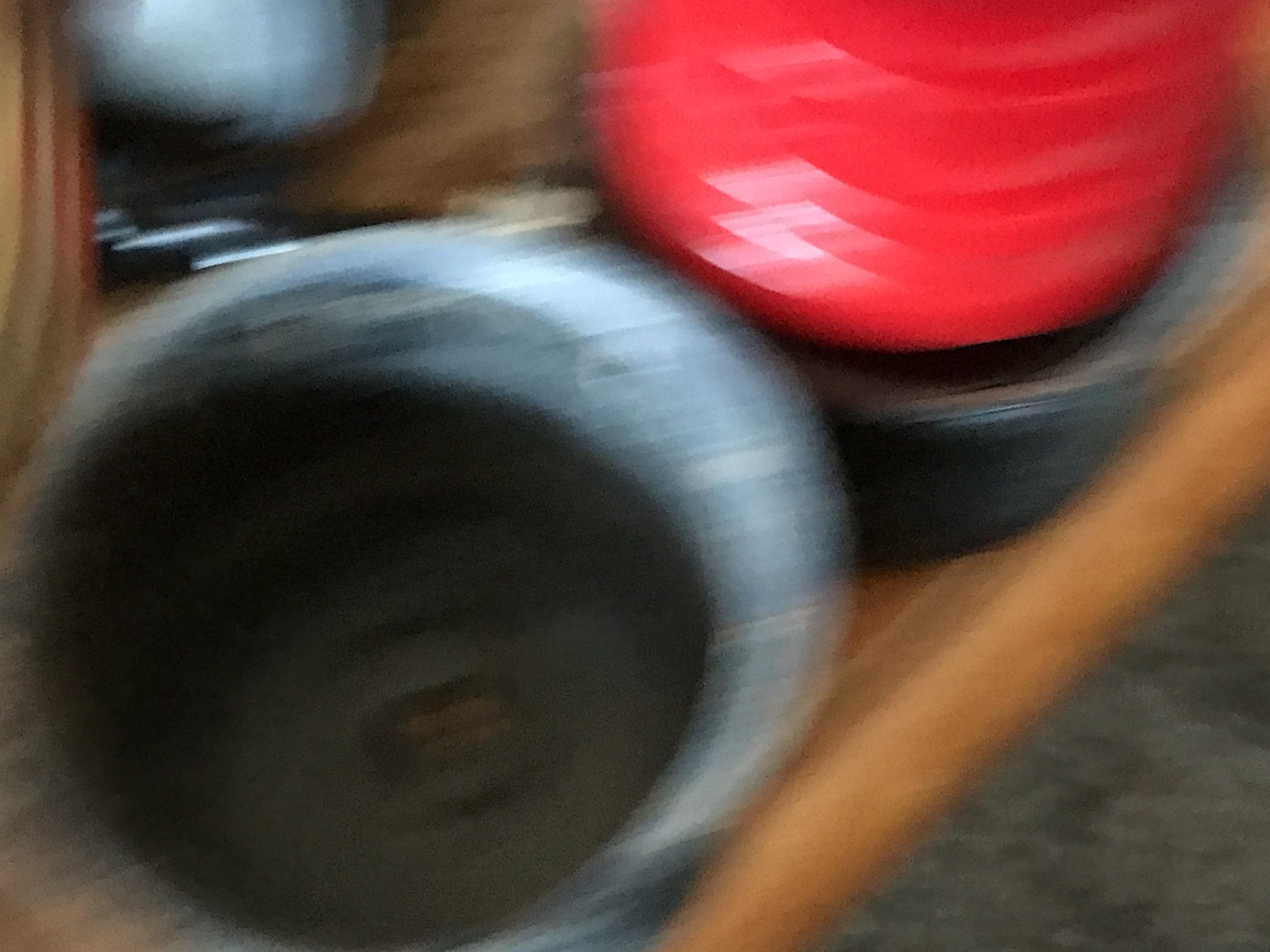This blurry, low-resolution image, possibly taken in motion, shows what appears to be a bird's eye view of two pots or buckets. The image, in a square format, has a white border and a mostly black interior. In the bottom left corner, a circular object can be seen, its interior black with a shiny upper right rim. Dominating the center and towards the top right, there is a dark navy-blue or black pot with a partially cylindrical red item on top of it. These objects rest on a light brown, woody platform, which may be a countertop or inside a wooden chest. The bottom right corner features a grayish patch, possibly the floor, suggesting the setting might be a garage or tool shed.